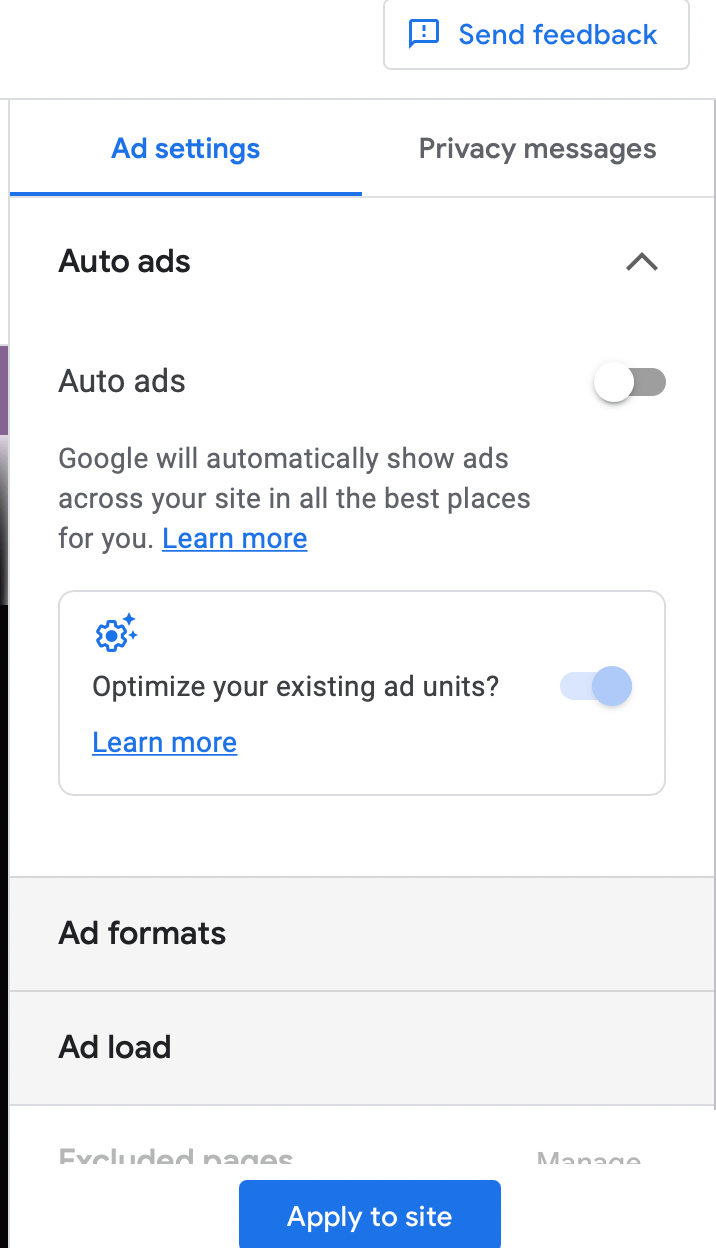A user navigates the ad settings on their Google Chrome Gmail app displayed on a phone screen. The interface has a clean, white background, accentuated by bold and colored text elements in black, gray, charcoal, and blue. The “Auto ads” feature is prominently highlighted with blue lettering, indicating it is toggled off, as the user prefers not to see automatic ads across their site. Below this, there is a gear icon accompanied by the text "Optimize your existing ad units," which is switched on. This section provides options for “Ad formats,” “Ad load,” “Apply to site,” and “Manage excluded pages.” Although an option for “Privacy messages” is present, it is underlined, signifying the current focus is on ad settings. To finalize changes, the user needs to apply the settings to the site using the button located at the bottom of the screen.